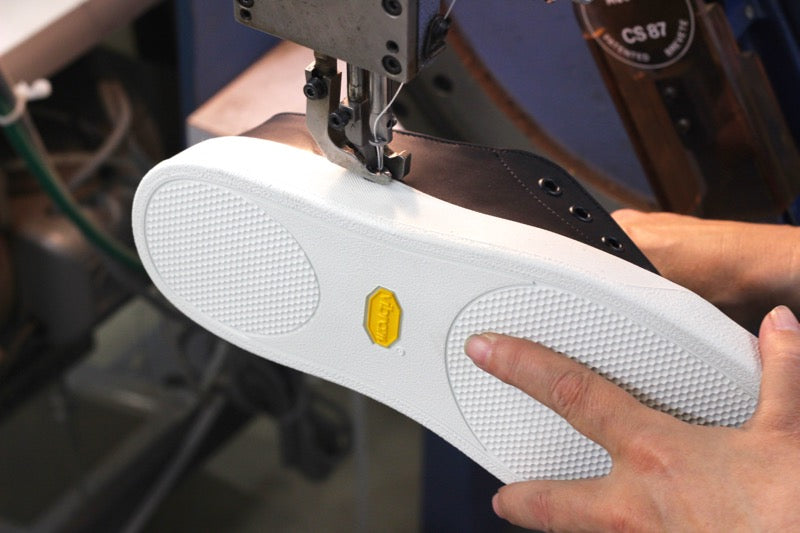A detailed photograph taken indoors depicts a Caucasian individual stitching a shoe using an industrial sewing machine made from thick, dark gray metal. The shoe, positioned on its side beneath the machine's footer, is primarily composed of black leather with a white rubber sole. The sewing machine is stitching white thread through the perimeter where the leather upper meets the sole. Notably, the shoe features tan stitching and black plastic eyelets for laces. At the center of the sole's bottom, a distinctive yellow, rectangular label—or octagonal insignia with a 'V' logo—is visible. Various parts of additional machinery, labeled "CS87" in the upper right corner, are partially seen in the blurred background.